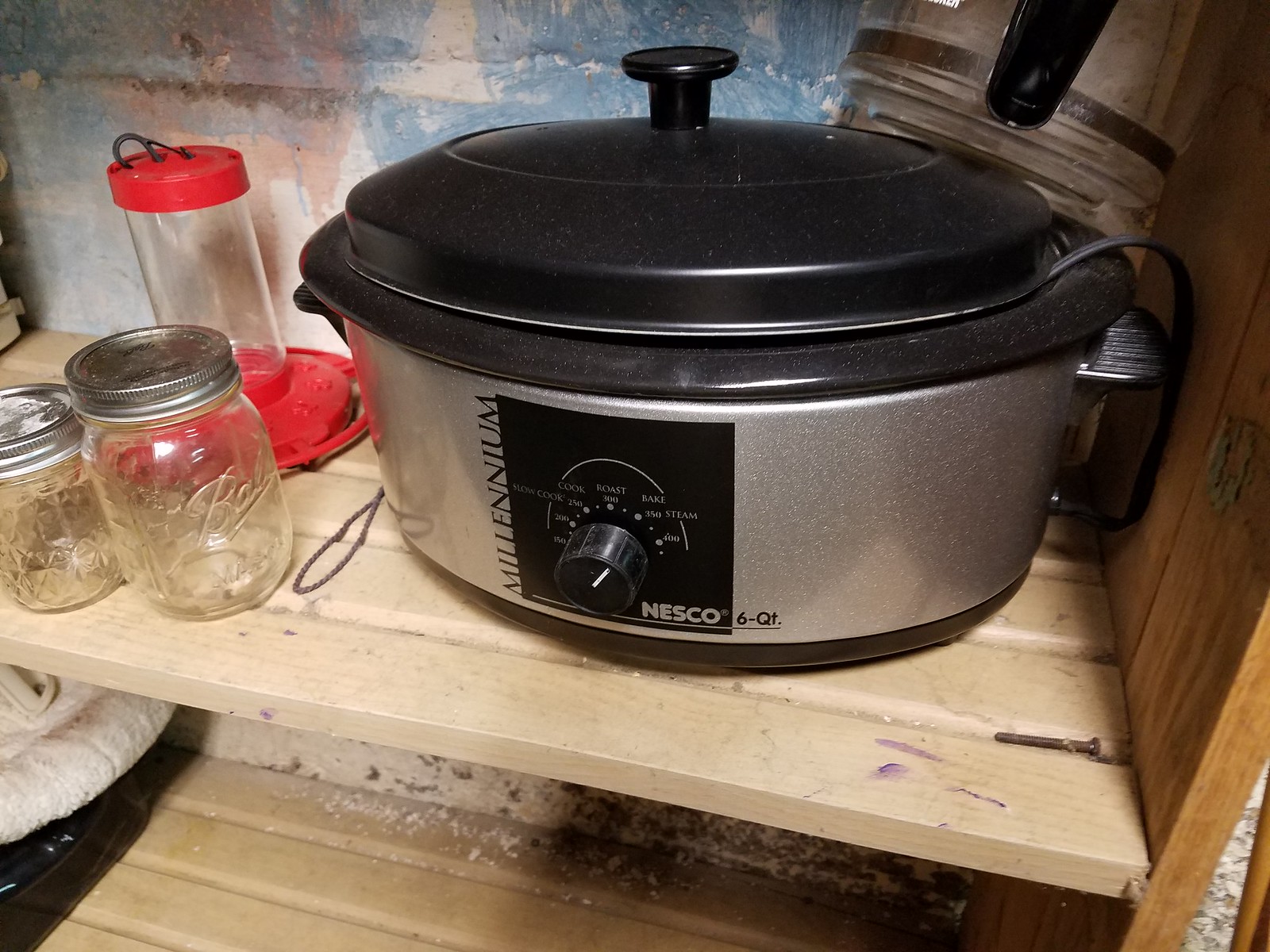This photograph showcases an oval-shaped electric slow cooker with a black lid and silver body, prominently featuring a Nesco logo. The cooker has a control dial with options for slow cooking, roasting, baking, and steaming, and various temperature settings ranging from 150 to 400 degrees Fahrenheit. The cooker sits on a wooden shelf with black handles and a black design on its top and bottom edges. Atop the cooker is a blender cup. To its left, two mason jars with silver caps are situated near a red hummingbird feeder with a clear bottom and a red top. The backdrop is a blue wall, and a brown string and nail are visible on the wooden cabinet.